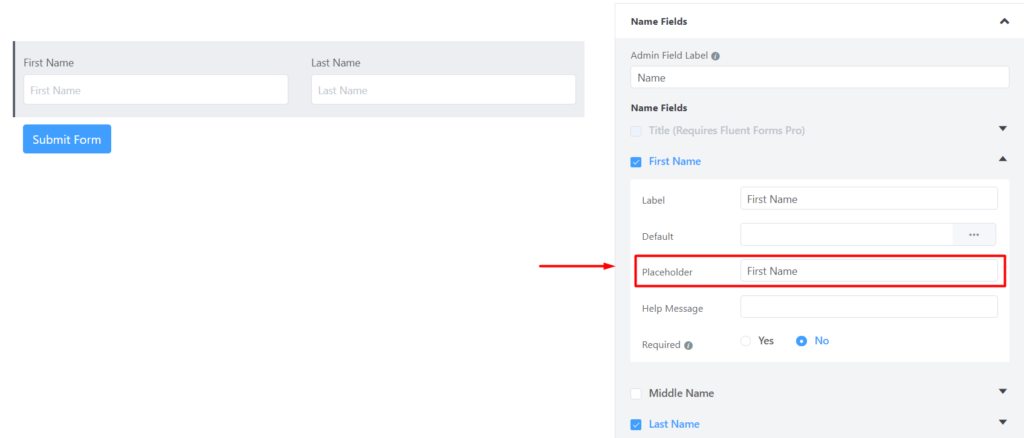A detailed screenshot captures a form submission interface predominantly set against a white backdrop. On the left side, a light gray rectangular section contains labeled fields: "First Name" above an empty white rectangular box for user input, and "Last Name" above another empty white rectangular box for entering the user's surname. Beneath these fields, set against the white background, resides a blue button labeled "Submit Form" in white text.

On the right side, a white header labeled "Name Fields" in black text features an upward arrow icon to the right. Below, in a gray section written in a slightly darker gray font, appears "Admin Field Label," followed by a white bar with "Name" inscribed within. Continuing down, a grayed-out icon indicates "Title (Requires Fluent Forms Pro)." In blue print, check marks appear next to "First Name" and "Last Name." The interface includes a series of editable sections: "Label" with "First Name" in the input box, "Default" with an empty white box for entries, "Placeholder" containing "First Name," and "Help Message" left blank. The "Required" field offers a yes or no option. Notably, the placeholder section is emphasized with a red arrow and rectangle. At the bottom, there are additional options for "Middle Name" and "Last Name," with "Last Name" being checked.